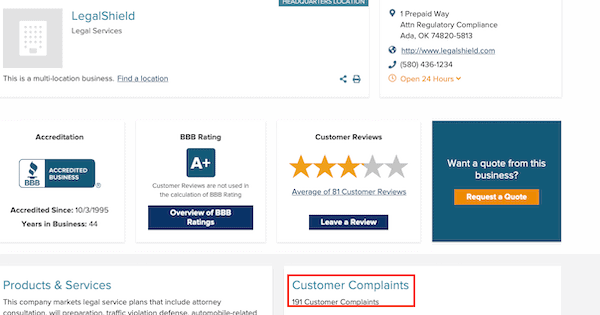In this detailed screenshot analysis, we observe the BBB listing for LegalShield, a company offering legal services across multiple locations, with an office based in Ada, Oklahoma. The searcher is evaluating LegalShield’s standing on the Better Business Bureau (BBB) website. Notably, LegalShield is BBB accredited, a certification they've held since October 3, 1995, denoting nearly 44 years of continuous accreditation and adherence to BBB standards. Their BBB rating sits impressively at A+, reflecting high standards of business practice over the decades.

However, this positive rating contrasts sharply with the customer reviews and complaints. The company has garnered 81 customer reviews with an average rating of just 3 stars, indicating a mix of customer experiences, many of which may not be favorable. Moreover, the screenshot, specifically highlighted with a red box, shows a concerning total of 191 customer complaints filed against the business. These complaints, despite the high BBB rating, suggest significant unresolved or untreated issues that could negatively impact customer trust and satisfaction.

The BBB page also features options to request a quote from LegalShield and explore additional products and services they offer, appealing to potential customers. However, the visible volume of unresolved complaints and mixed reviews could serve as a red flag for prospective clients, signaling areas where LegalShield might need to improve transparency and customer service.